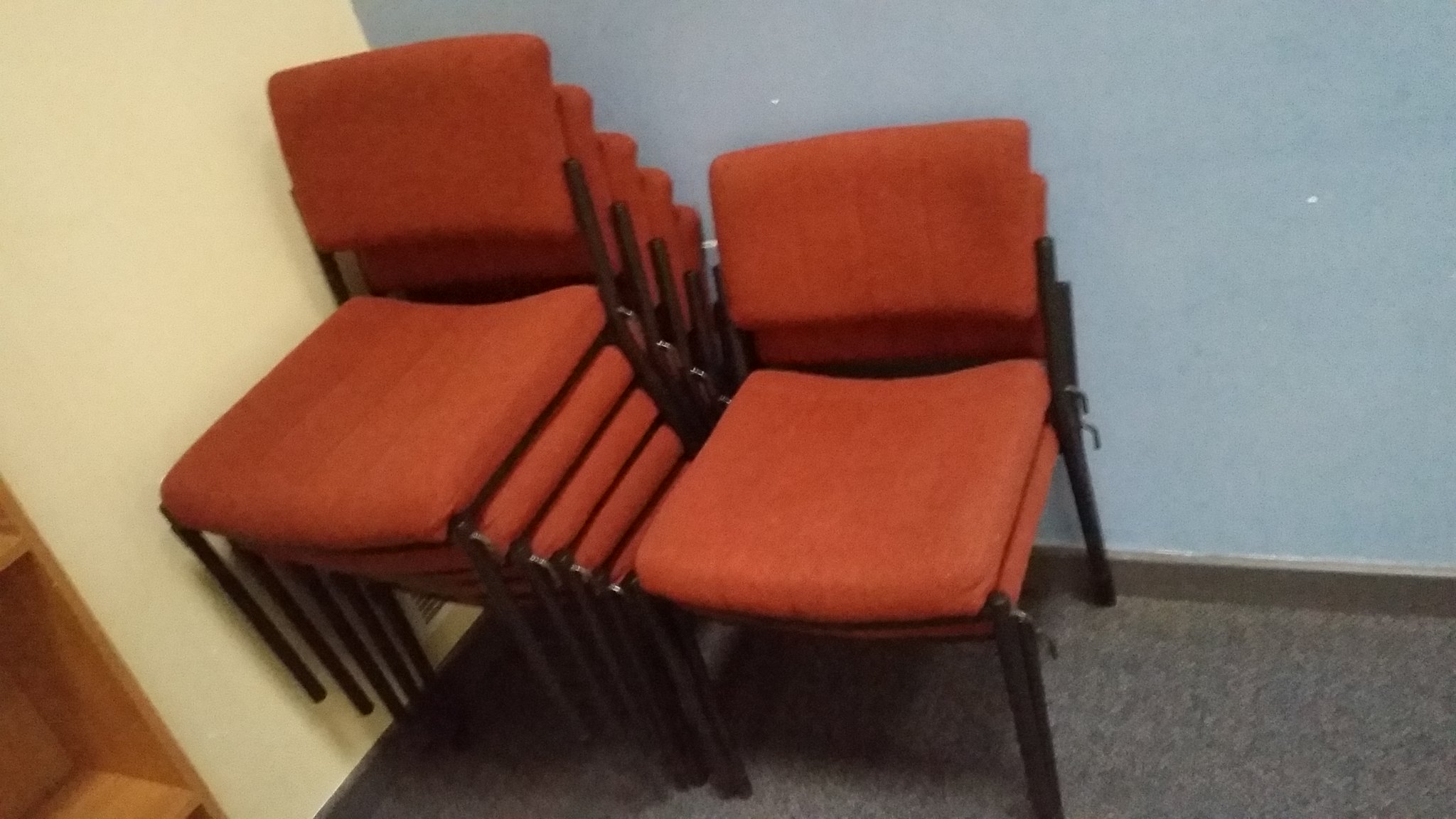The indoor digital photo depicts a somewhat blurry scene of two stacks of burnt orange fabric chairs with black metal legs, situated in the corner where the beige left wall and a light blue back wall meet. The back wall appears to have some missing chunks of paint revealing white patches. The floor is covered in office-style short multicolored blue carpet bordered by a gray baseboard. The stack on the right consists of two chairs, while the stack on the left has four chairs. There is a small tan wooden structure, possibly a bookcase, in the bottom left part of the photo. The chairs have a distinctive design with a space separating the back and the seat, which are both upholstered in the same burnt orange fabric.